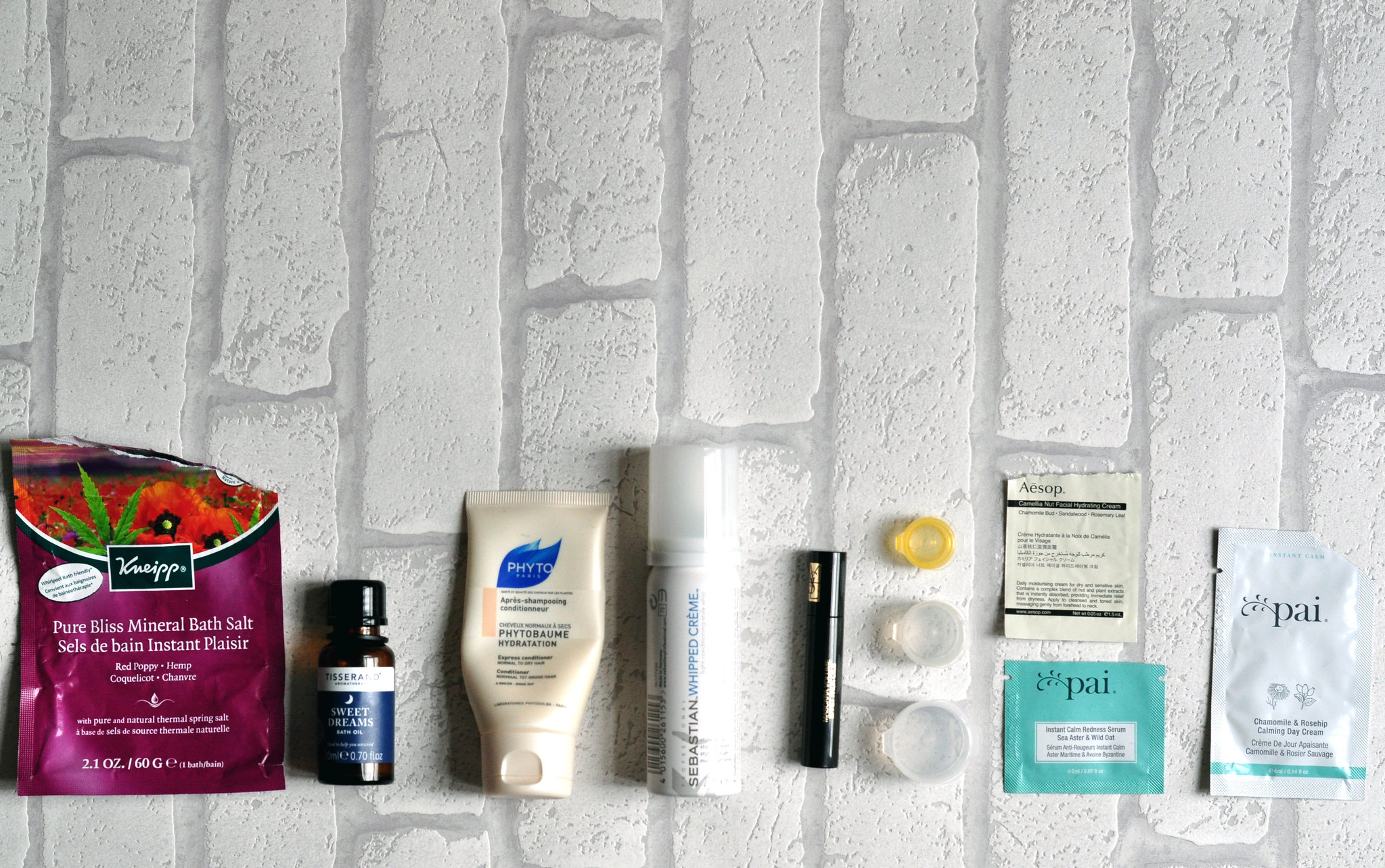This captivating image displays an eclectic collection of skincare products, meticulously arranged on a white brick surface, which despite its cracks and worn appearance, serves as an intriguing backdrop likely mimicking a dorm room or military housing floor. The assortment of 11 items presents a diverse range of beauty and wellness solutions. 

From left to right, the first item is an opened magenta pink bag labeled "KNEIPP," containing "Pure Bliss Mineral Bath Salt" with red poppy and hemp, weighing 2.1 ounces (60 grams). French descriptions reiterate its contents and benefits. Next, a brown bottle with a black lid bears the name "Tisserand" (suggesting a blend of terms "Tisser" and "Therapy") and features a dark blue label indicating "Sweet Dreams" oil, in a volume of 0.7 fluid ounces. 

Following this is a cream-colored bottle adorned with a blue leaf logo and the brand name "Phyto." It appears to be an après-shampoo conditioner emphasizing "Phytojoba Hydration." Further along is a container resembling a whipped cream bottle, boldly labeled "Sebastian Whipped Crème," suggesting a luxurious facial cream. 

Adjacent is a sleek, black, mascara-sized tube with unreadable text, intriguing yet mysterious. Three consecutively placed contact lens cases—yellow small, medium white-clear, and large white-clear—provide a curious juxtaposition next to the skincare items. To the right, two small packets lie, one opened and labeled "ASAP," with unseen detailed text. Below rests a green sample packet from "PAI," promoting "Instant Calm Redness Serum" with sea aster and wild oat extracts.

The final product, also from "PAI," is a predominantly white sample packaging adorned with plant illustrations, denoting "Chamomile and Rosehip Calming Day Cream," with bilingual descriptions in French. This array showcases a thoughtful curation of skincare and alternative health care products, catering to diverse beauty and wellness needs.